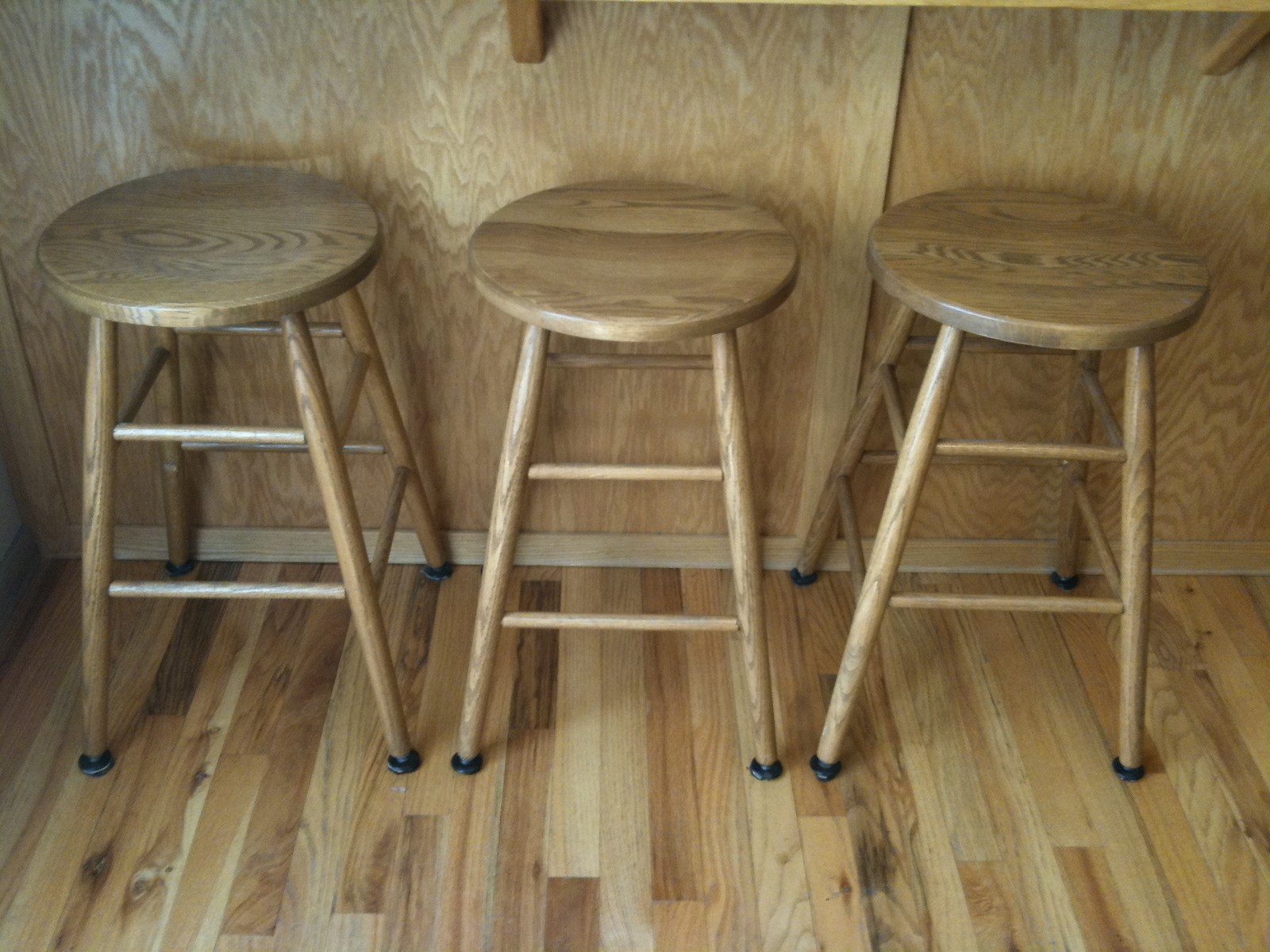This color photograph, bathed in bright natural or artificial lighting, showcases three wooden bar stools standing side-by-side against a matching wooden wall. Both the floor and the wall exhibit distinctive wood markings and designs, evoking a warm reddish-brown tint that permeates the entire image. The stools, each featuring a round top and no backrest, are constructed of solid wood with a coat of clear protective finish. Each stool has four legs, fitted with black rubber grips to prevent floor scratching, and is interconnected by two sturdy cross rungs. They are set in a neat line on a narrow plank wooden floor, which varies in color and grain pattern, running vertically from the bottom to the center of the frame. Above the stools, a partially visible shelf or countertop made of plywood adds to the natural wooden ambiance of the scene.